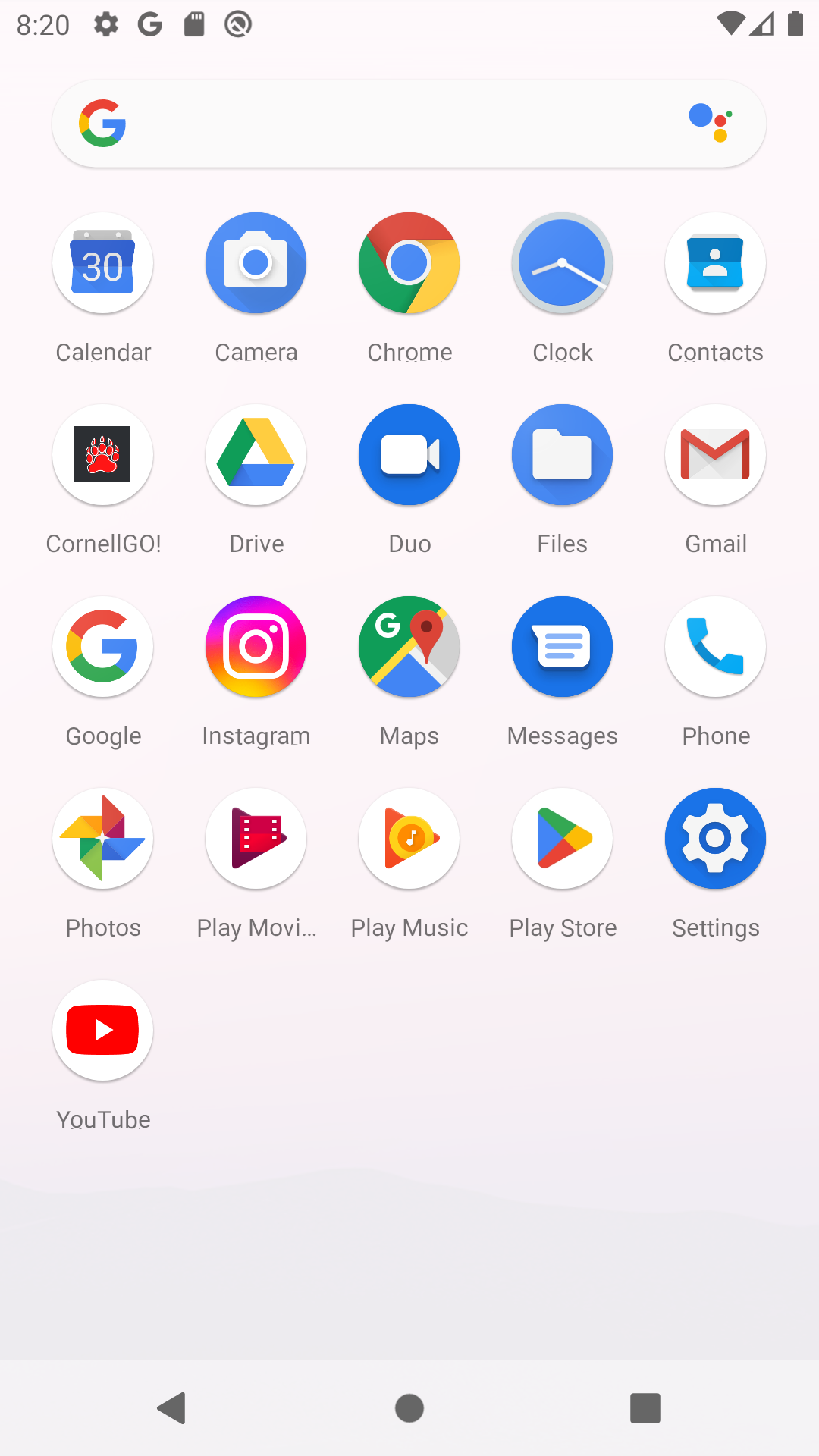The image depicts the app drawer of an Android device, which could either be a wide phone or narrow tablet based on its dimensions. The background is predominantly gray, highlighting the simplicity of the interface. At the top, there is a search bar, followed by a grid of app icons. The pre-installed apps present include Calendar, Camera, Chrome, Clock, Contacts, Drive, Duo, Files, Gmail, Google, Maps, Messages, Phone, Photos, Play Movies, Play Music, Play Store, Settings, and YouTube. In addition, three user-installed apps—Cornell, Go, and Instagram—are also visible. The Cornell app likely serves as a student portal for Cornell University. 

Notably, all app icons are displayed with a uniform circular background. At the bottom of the screen, traditional Android navigation buttons—back, home, and recent apps—are visible, indicative of an older Android version. The notification area at the top of the screen shows a middling percentage of notifications, a fully charged battery, and a strong Wi-Fi connection.